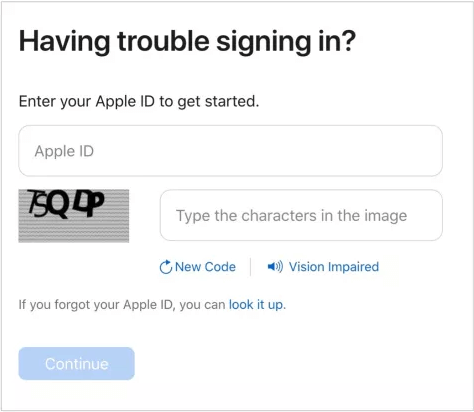This image depicts a user interface for recovering an Apple ID. At the top, bold black text reads, "Having trouble signing in?" followed by the instruction, "Enter your Apple ID to get started." Below this text is a field labeled "Apple ID," prompting the user to input their identity credentials. Further down, there are instructions to type the characters shown in an image to the left into a verification field. The characters displayed are "TSQBP," all in uppercase letters. There are also options to request a new code or to select an alternative process for visually impaired users. Additionally, a link is provided for users who have forgotten their Apple ID and need to look it up. The color scheme includes a white background with black and blue text, and the "Continue" button is highlighted in a blue dialogue box located at the bottom left corner of the interface.